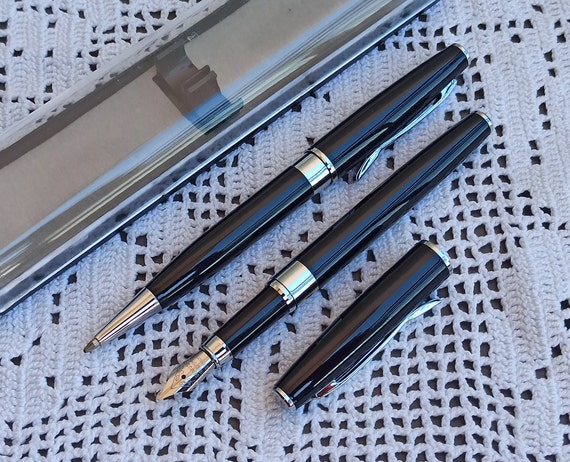The image showcases a luxurious pen set displayed on a white, doily-patterned knit tablecloth with visible holes, set against a darker surface table. Positioned diagonally at the top of the image is a transparent plastic case with a gray bottom, which originally held the pens. Below the case are two glossy black pens arranged diagonally, one above the other.

The top pen features a traditional fountain pen design with a removable black cap adorned with a silver ring and a silver clip, allowing it to be attached to a pocket. The pen's center also has a silver metal section, contributing to its elegant appearance.

The pen below it is distinguished by its triangular, spearhead-like nib, resembling those used in traditional dip-and-ink pens. This pen also has a silver band slightly below the midway point. The cap for this pen, also black with a silver ring, lies beneath it.

Both pens are evidently part of a high-end set, with the sophisticated presentation on the delicate doily further enhancing their luxurious feel.